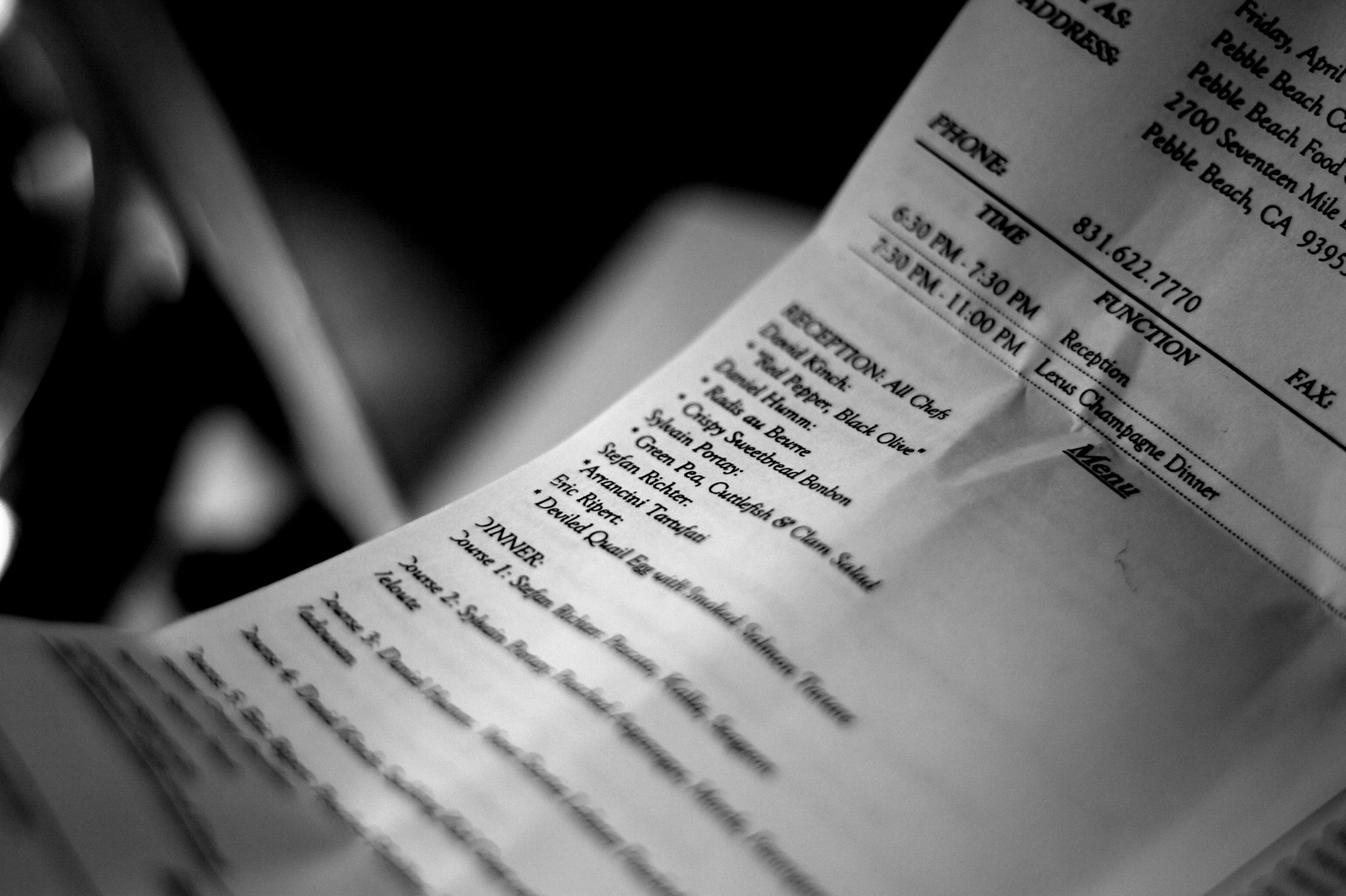This detailed close-up image depicts the central portion of a white paper, partially blurred on the sides, making some parts difficult to read. The paper outlines an event schedule and menu for a reception and a Lexus Champagne Dinner held at Pebble Beach, California, with the contact phone number 831-622-7770. It details the event times: 6:30 PM to 7:30 PM for the reception, and 7:30 PM to 11:00 PM for the dinner. The visible menu items include:

- **Reception Menu:**
  - David Kinch: Red Pepper, Black Olive
  - Daniel Humm: Radish au Beurre, Crispy Sweetbreads Bon Bon
  - Sylvain Portet: Green Pea Cuttlefish and Clam Salad
  - Stephan Richter: Arancini, Tarta Fati
  - Eric Ripert: Deviled Quail Egg with Smoked Salmon 

The dinner courses are mentioned but are too blurry to read clearly. The left side of the image contains a lot of black space with indistinguishable white objects due to the blur, likely adding contrast to the clear central text.